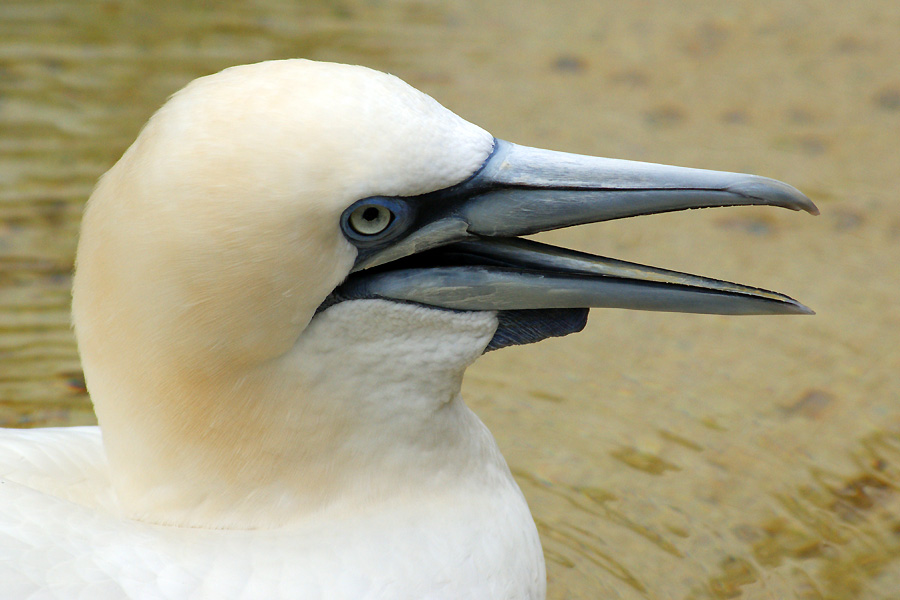This highly detailed photograph captures a striking close-up side-profile of a white bird, revealing its fascinating features as it floats on murky, light brownish-green water. The bird's pristine white feathers, which look as soft as cotton, contrast sharply with its intriguing beak and eye markings. The beak, an undamaged, grayish hue with a subtle black outline, extends impressively close to the bird's eye, which is encircled by a dark gray ring and outlined in blue, suggesting perhaps an albino or unique species. The bird's beak is open, possibly indicating it is making a sound or being fed at the moment the snapshot was captured. Ripples in the water extend outward, indicating movement and contributing to the dynamic nature of the scene. The image, set in an outdoor environment during the day, showcases the bird looking sideways to the right, with its beak and gaze directed rightwards, embodying a peaceful moment amidst the seemingly muddy waters of what could be a lake, pond, creek, or swamp.